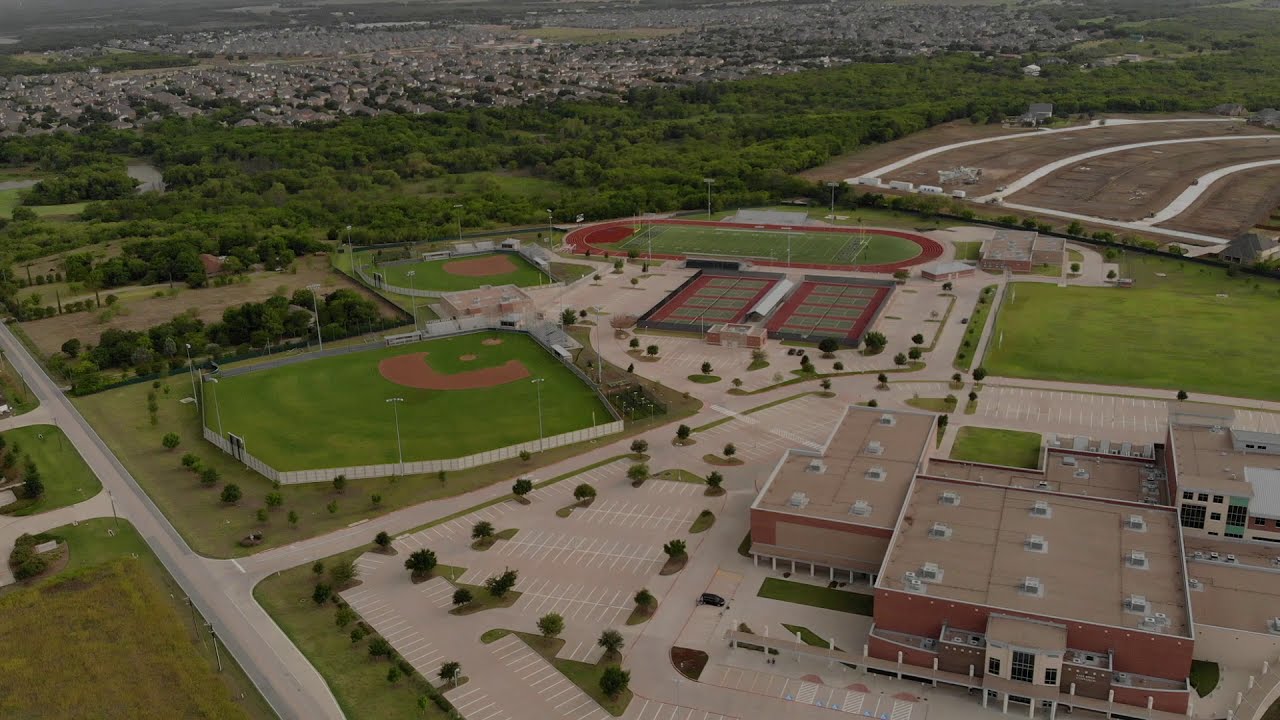This horizontally rectangular, full-color aerial photograph was captured outdoors during the daytime, likely from a small plane. Centered in the image is a school complex surrounded by a variety of athletic facilities including several tennis courts, a football field encircled by a track, and two baseball diamonds. Three or four brown buildings with flat roofs and white air conditioning units on top are also visible. The upper left portion of the image reveals a town with numerous residential homes and some wooded areas. The photograph brims with hues of red, brown, green, black, white, tan, yellow, and orange, and lacks any visible text or borders.